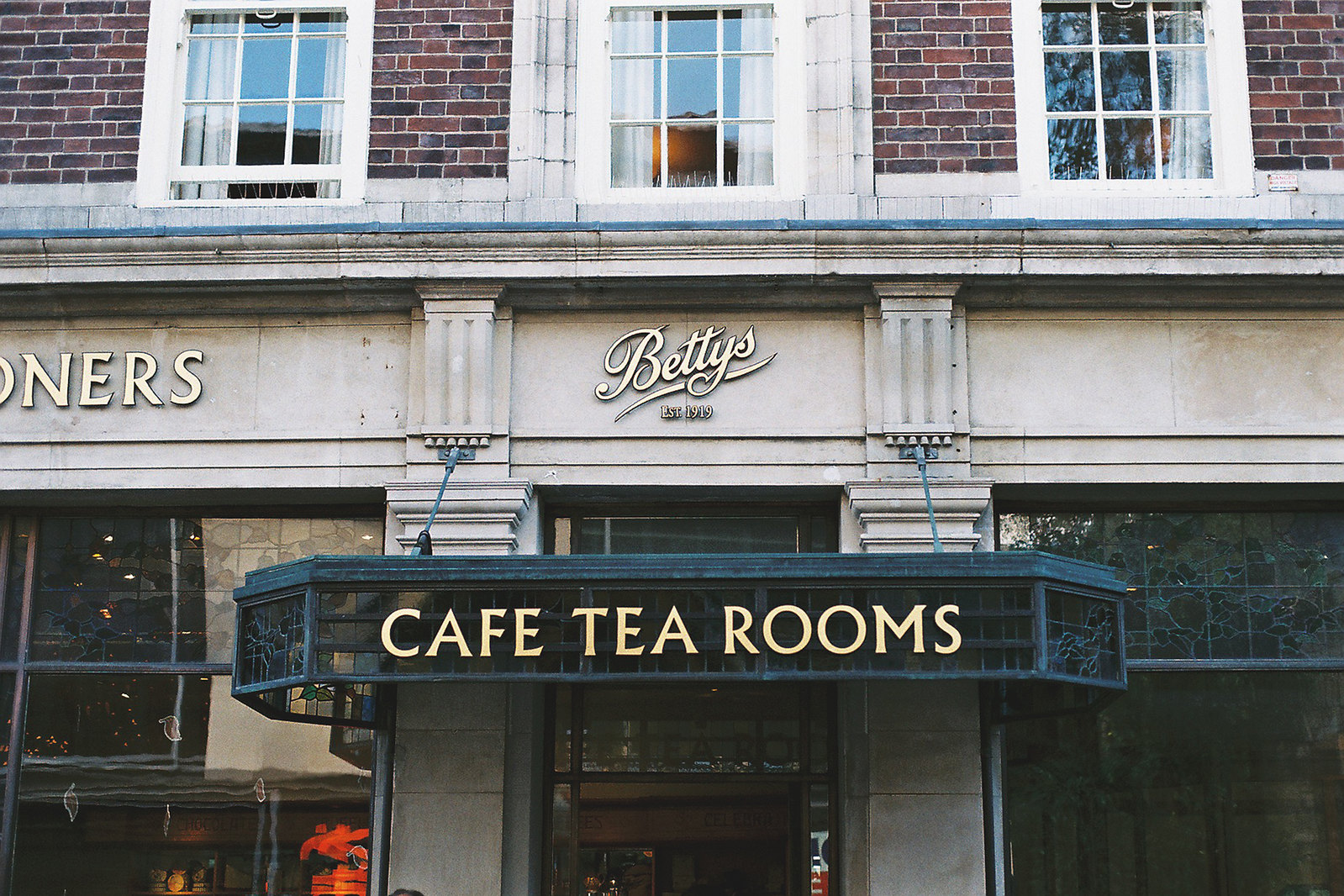The photograph captures the front entrance of Betty's, an elegant establishment founded in 1919. The image showcases a brick building with vintage Victorian-style architecture. The facade features a notable gold script sign that reads "Betty's, E.S.T. 1919," affixed to the wall above the entrance. Adjacent to this, partially visible letters "O-N-E-R-S" are seen on the wall. Below the main sign, an ornate hanging sign adorned with stained glass and gold letters spells out "Cafe Tea Rooms."

The lower portion of the building includes large glass windows, allowing glimpses into the warmly lit interior. The doorway, centrally located, is flanked by the columns which support the marquee. The upper half of the structure consists of red bricks and three white-framed windows with white curtains, adding a touch of refinement. Additionally, the middle window exhibits an orange glow, likely from an interior light, enhancing the inviting atmosphere. The architecture reflects vintage charm with bluish-green tarnished copper elements, especially around the marquee and columns, contributing to the building's historical and timeless appeal.